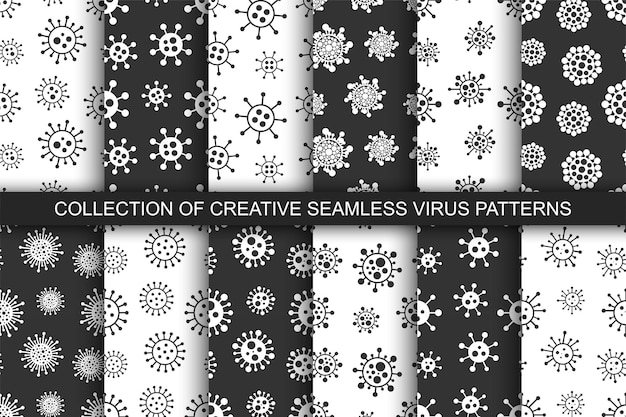The image is a detailed black-and-white composition displaying a collection of various seamless patterns, all inspired by the visual structure of viruses. The alternating designs are meticulously arranged with sections featuring a white background adorned with black circular virus motifs, and other sections showcasing a black background with the reverse pattern in white. Each virus-like shape consists of a central circle with lines extending outwards, some terminating in small dots or balls, giving a repetitive and organized feel to the patterns. The center of the image is highlighted by a black rectangle stretching from left to right, which reads, "Collection of Creative Seamless Virus Patterns." This array is reminiscent of fabric swatches arranged as they might be in a fabric store, each piece either predominantly white or black. The patterns overlap slightly, enhancing the cohesiveness of the collection.